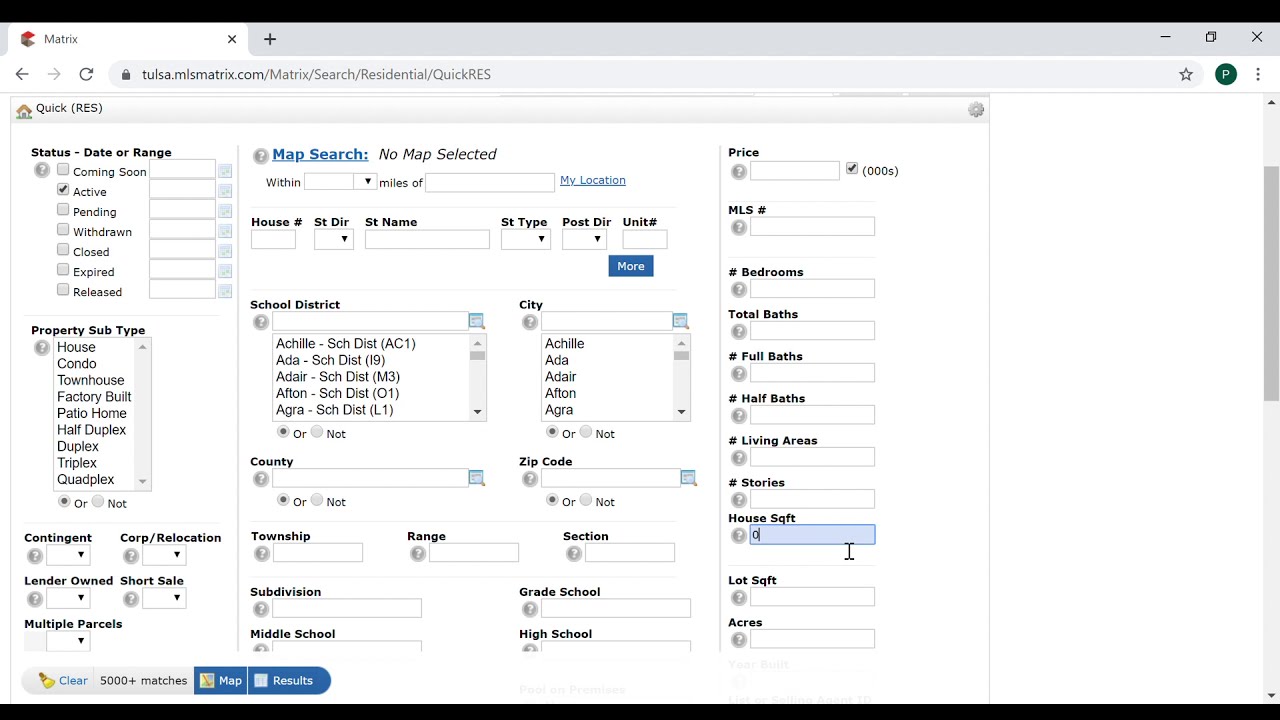This screenshot shows a detailed view of a web page from tulsa.mlsmatrix.com/matrix/search/residential/quick res. The page is primarily white with a thin black header and footer, along with some gray accents. At the top of the page, the word "MATRIX" is in tab, and below, a white bar labeled "Quick (Res)" is accompanied by a home icon.

The interface features numerous forms and filtering options arranged in a structured layout, allowing users to perform detailed searches for properties. On the left side, various forms are organized under sections such as "Status" (including options like 'Active'), "Date Range," and "Property Subtype" (offering choices like house, condo, townhouse, factory-built). Other categories on this side include contingent statuses, corporate relocations, lender-owned properties, and short sales.

In the middle section, there's a "Map Search" feature in blue text, currently indicating "No map selected." This is followed by fields for further refining searches with house number, street direction, street name, street type, school district, city, county, zip code, township, range, section, and subdivision criteria.

Over to the right, additional filters allow users to specify the desired price range, MLS number, number of bedrooms, bathrooms (full and half), living area, and acreage. Other search criteria include school options for various education levels (grade, middle, high), and multiple parcels. This level of detail and customization supports comprehensive property searches for both residential and commercial real estate needs.